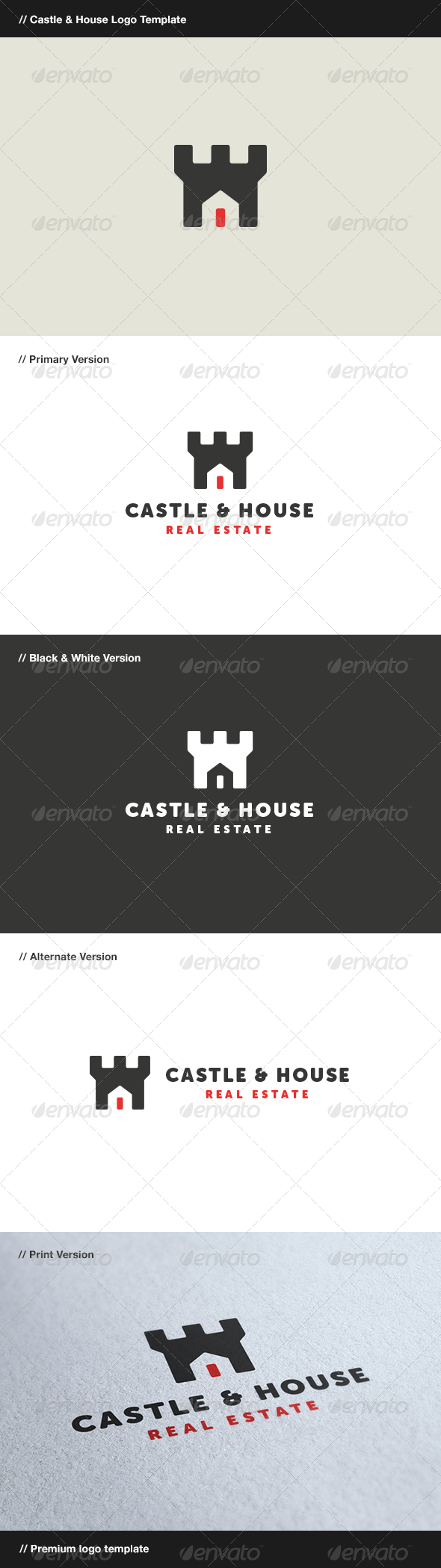The image depicts a vertically arranged sequence of five placards, each progressively differing in design elements but unified by the Castle House Real Estate logo. Starting from the top, the first placard features a light gray background with a simplistic black castle logo and a small red door. The second placard presents the same logo on a white background with the text "Castle House Real Estate" beneath the castle. The third placard showcases a black background with a reversed color scheme—a white castle with a white door and the text "Castle House Real Estate" in white. The fourth placard, labeled as the "Alternate Version," again has a white background but emphasizes the text differently: "Castle House" in black and "Real Estate" in red. Finally, the bottom placard, referred to as the "Print Version," rests on a blue-gray background, featuring the same black castle with a red door and the text "Castle House Real Estate" in black with "Real Estate" slightly smaller and in red. Each placard demonstrates a consistent branding theme with minor variations, contributing to a cohesive yet dynamic visual presentation.